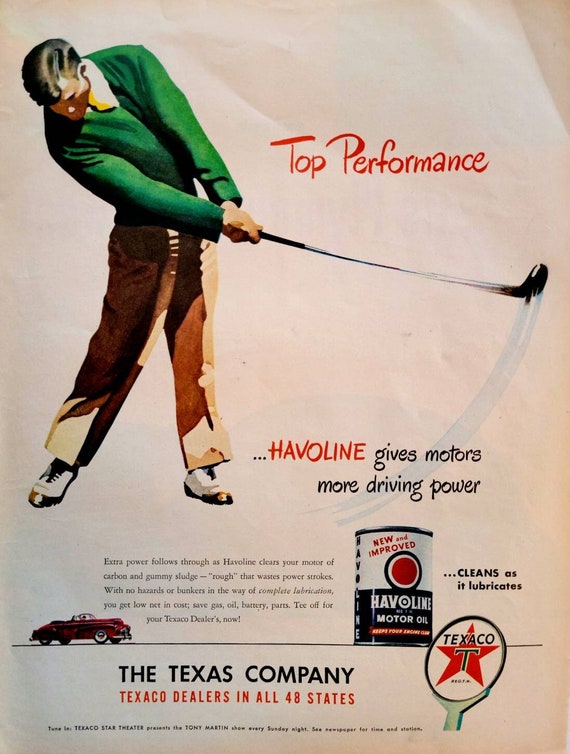This vintage advertisement poster for Havilene Motor Oil likely once adorned a gas station or car service center. The ad prominently features a detailed drawing of a man in a green sweater, tan pants, and golfing shoes, swinging a golf club. The text at the top boldly declares "Top Performance" in red letters, linking the golfer's success to the product's quality. Centered in red letters is "Havilene," with the slogan "Havilene gives motors more driving power" below it in black. The ad emphasizes the product's benefits with a small image of a motor oil can that reads, "New and Improved Havilene Motor Oil – Cleans as it Lubricates."

In the lower right corner, the familiar Texaco service station logo is displayed, featuring a black "T" encircled by a red star. Adjacent to this is a small depiction of a 1950s-era red convertible, reinforcing the automotive theme. Along the bottom, the text notes, "The Texas Company, Texaco dealers in all 48 states." The background of the advertisement is a warm peach color, tying the various elements together. The overall design cleverly associates the precision and excellence of golf with the superior performance of Havilene Motor Oil.